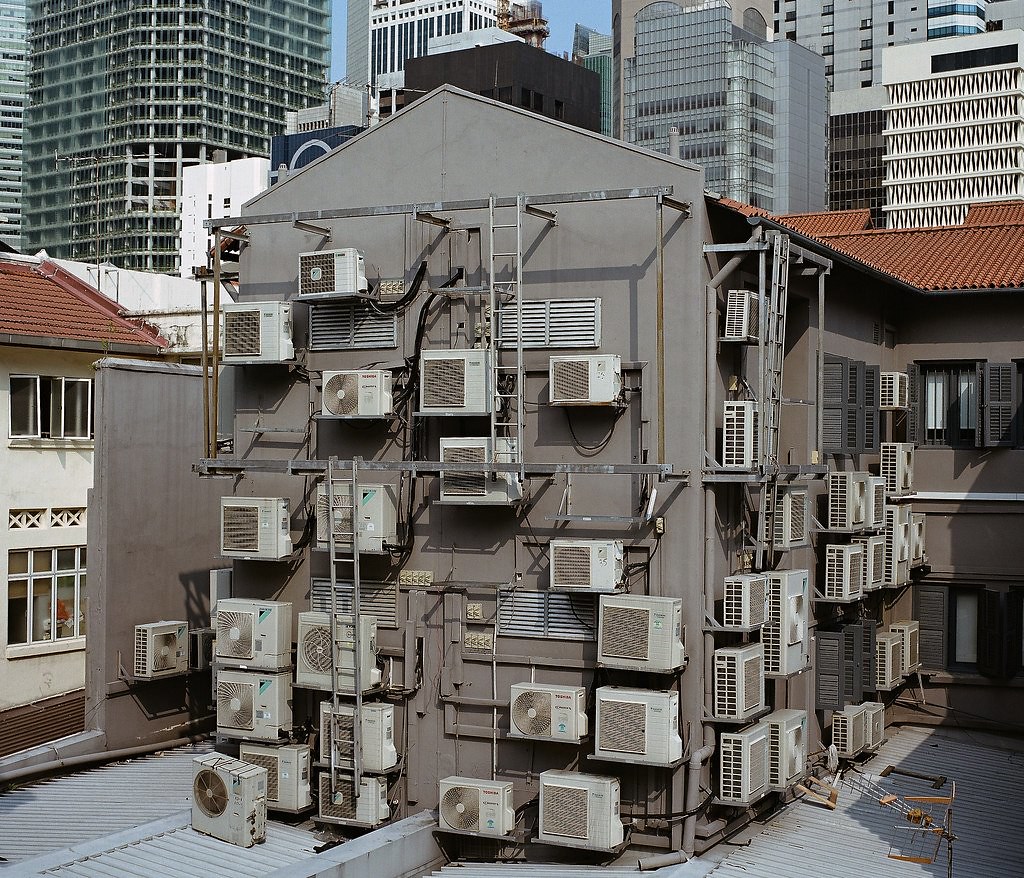The image depicts the rear side of a large building with gray walls, bristling with numerous air conditioning units. At least 20 classic grayish-white air conditioner units, some of varying brands, are attached to the exterior, with even more visible on the adjacent wall. This setup dominates the back of the building. Two ladders are seen: one rising from the ground to the second level of beams, and another, about two meters higher, leading to the top of the second beam. There are white-curtained windows interspersed among the units. Behind this structure, a residential-looking building with a red roof contrasts against the gray walls. In the backdrop, you can see several tall, clean-looking skyscrapers with many windows, emphasizing the city's urban landscape.